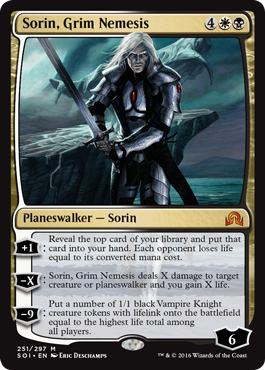The dark-themed card in question appears to be a character or informational card, prominently featuring elegant gold trim within its borders. At the top, the name "Sorin, Grim Nemesis" is prominently displayed, with the number "4" situated nearby, indicating its mana cost.

The central feature of the card is a highly detailed depiction of the character Sorin. He is showcased wearing imposing armor adorned with a central red gem on the chest plate, as well as additional red gems on the shoulders, which appear to be embedded in the armor. Sorin's appearance is striking, with his flowing white hair cascading down and a cape billowing behind him, adding to his commanding presence. In his hand, Sorin clutches a formidable sword, emphasizing his readiness for combat.

The card specifies Sorin's type as "Planeswalker - Sorin" and provides an array of abilities and effects. One of the abilities states, "Reveal the top card of your library and put that card into your hand. Each opponent loses life equal to its converted mana cost." Another ability indicates, "Sorin, Grim Nemesis deals X damage to target creature or Planeswalker and you gain X life," where "X" is a variable dependent on Sorin's loyalty counters. Additionally, the card offers a powerful ultimate ability: "Put a number of 1/1 black Vampire Knight creature tokens with lifelink onto the battlefield equal to the highest life total among all players."

Finally, at the bottom of the card, the number "6" is displayed, signifying Sorin's initial loyalty counters when he enters the battlefield. This comprehensive and visually captivating card clearly delineates Sorin's formidable abilities and his distinct role in the game.